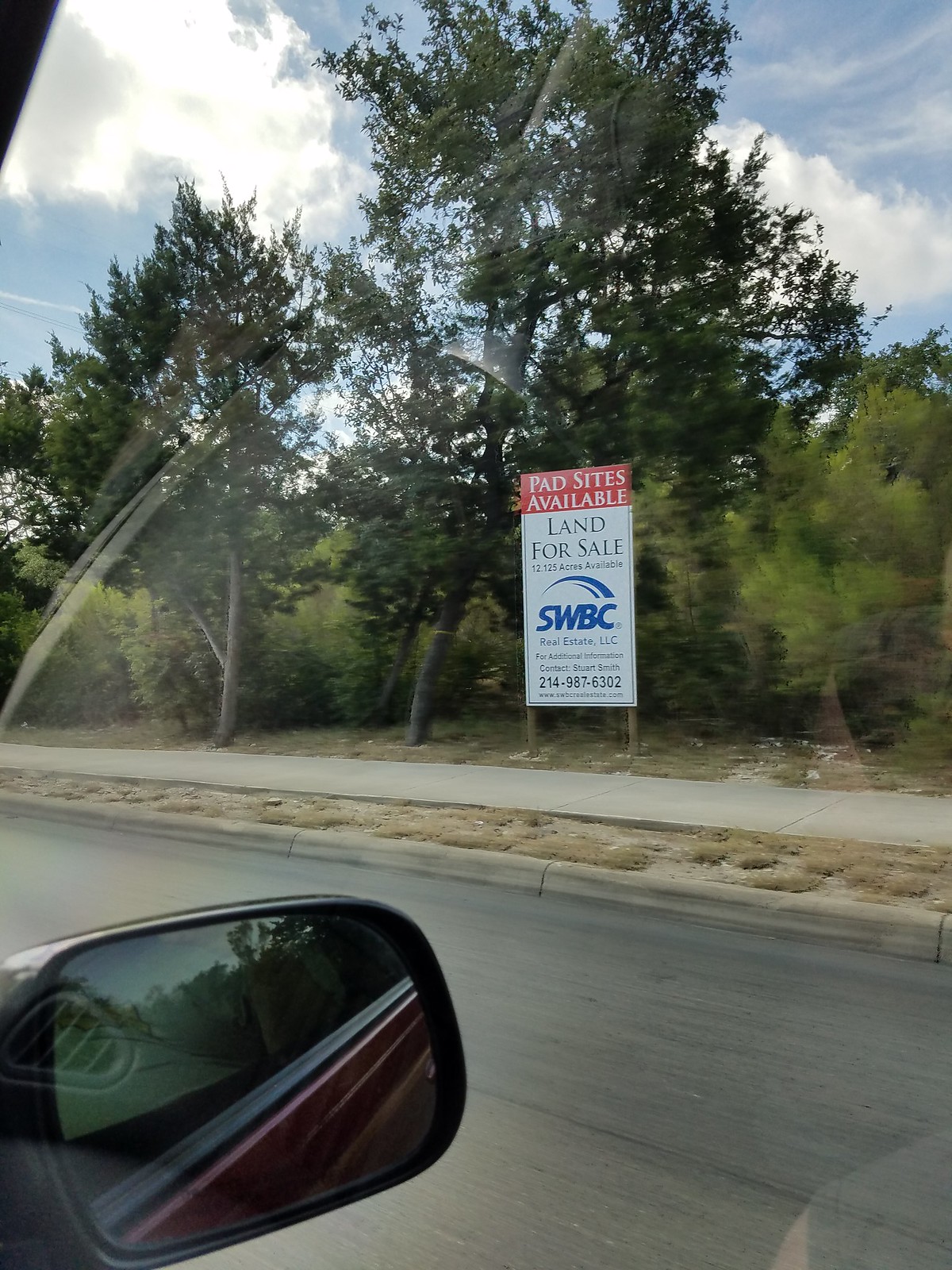Through the passenger window of a moving car, this image captures multiple reflective elements and scenery outside. The window itself shows some slight glare and reflections, including a glimpse of the car's side mirror. In the mirror, we can see a portion of the car's exterior and a heavyset individual seated in the passenger seat. The car appears to be traveling on an asphalt road, adjacent to a cement curb and sidewalk. The sidewalk borders patches of very dry soil, with a row of trees visible further in the background. Prominently visible is a large, white sign held up by metal stakes, advertising "Land for Sale" by realtor SWBC. A red banner across the top of the sign reads "PAD sites available" in clear lettering.